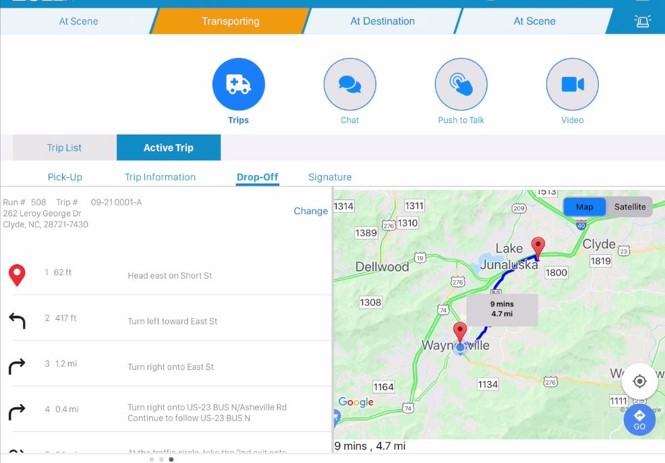Screenshot of a Travel Search Interface

The screenshot displays a travel search interface with a dominantly white background. At the top, there's a blue bar with four menu tabs extensively arranged: "At Scene," "Transporting," "At Destination," and "At Scene" again, with the "Transporting" tab highlighted in orange, indicating its selection.

Just beneath the menu bar are four distinct buttons, each representing a different feature:
1. A blue-highlighted button with a white ambulance icon labeled "Trips."
2. A grayed-out circle with two blue chat icons labeled "Chat."
3. A grayed-out hand pressing a button symbol titled "Push to Talk."
4. A grayed circle displaying a blue video icon under the title "Video."

Following these buttons are two rectangular options: "Trip List" and "Active Trip," with "Active Trip" currently activated.

The interface is divided into two main columns. The left column is dedicated to travel progress:
- The first field is "Pickup," providing specific trip details, including the Pickup address.
- The second field, "Trip Information," outlines the trip's data.
Below these fields, there are icons depicting travel activities, featuring a red downward location arrow and directional arrows denoting left or right turns. The distance calculator is strategically placed between each travel stage.

The right column contains the map. This colored map, framed in green and white, distinctly marks highways with numbers like 1314, 1311, 1389, and 1310, presumably indicating exits, alongside three main cities: Waynesville, Junaluska, and Clyde. In the upper corner of this section are two buttons: a blue-highlighted "Map" button and a grayed-out "Satellite" button. Down further, two blue round buttons appear: the first is a blue-highlighted "Go" button, and the second carries a navigation icon. 

At the bottom of the map, travel time and distance are clearly indicated: 9 minutes and 4.7 miles, respectively.